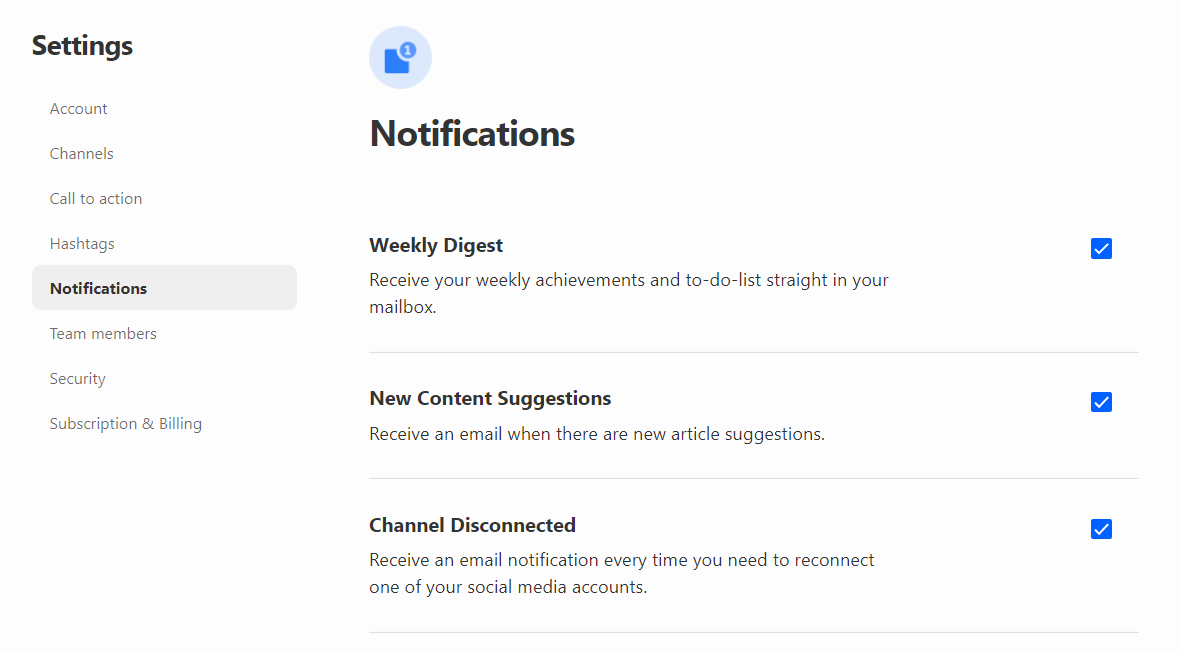The image depicts a settings page with a minimalist design, primarily using shades of white, gray, black, and blue. On the left-hand side, there is a vertical menu set against a white background. The heading "Settings" is prominently displayed in black bold text. Underneath this heading, the following menu items are listed in gray: 

- Account
- Channels
- Call to Action
- Hashtag
- Notification
- Team Members
- Security
- Subscription and Billing

A bolded "Notifications" text denotes the active menu item. Next to "Notifications" is a gray bar or rectangle highlighting it as the selected option.

Moving to the right and slightly upwards on the page, there is a circular icon with a square in its center, marked with the number "1" at the upper right corner. This icon is shaded in varying hues of blue, from light to dark.

Below this icon, the page content begins with the heading "Notifications" in bold. The first section is titled "Weekly Digest" with the description, "Receive your weekly achievements and to-do list straight in your mailbox," accompanied by a blue checkbox on the far right, indicating it is enabled.

Following this, another section reads "New Content Suggestions" with the description, "Receive an email when there are new articles suggested." Again, a blue checkbox on the far right signifies that this option is enabled.

The final section in the notifications settings is "Channel Disconnected," described as "Receive an email notification every time you need to reconnect one of your social media accounts." Like the previous options, this section includes a blue checkbox on the far right, also marked as enabled.

The overall page maintains a clean and organized aesthetic with a consistent color scheme of white, gray, black, and shades of blue.